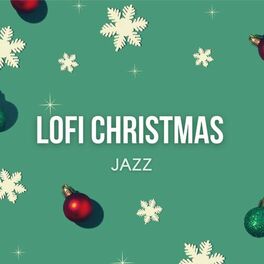This image is a likely album cover or flyer for "LOFI CHRISTMAS JAZZ." The perfectly square image has a turquoise, jade green background, scattered with white snowflakes and red bulb ornaments. At the center, in bold white all-capital letters, it reads "LO-FI CHRISTMAS," with "JAZZ" in smaller white letters beneath. More red ornaments decorate the bottom, and a green ornament appears in the lower right-hand corner. The clean, minimalistic design features only these elements on the greenish-blue backdrop.